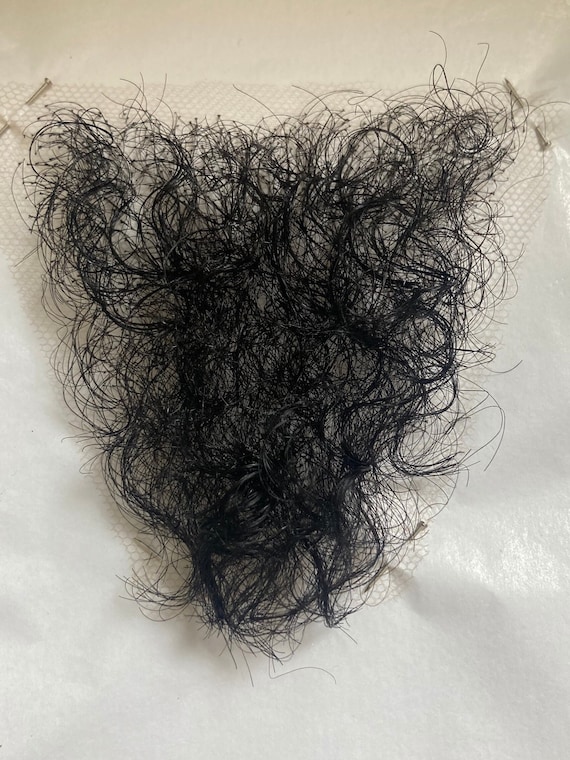The vertically rectangular, full-color photograph primarily showcases a large wad of black, curly hair arranged in an upside-down, equilateral triangle shape. It lies on a white surface that resembles a paper towel, although the precise material is unclear. The hair is pinned at the upper left and upper right corners by two pins or nails. The background is stark white, contributing to the bright and clearly lit setting of the image. There are no additional objects or text present, making the focus solely on the hair, which at first glance might be mistaken for a woman's pubic hair due to its shape and appearance.